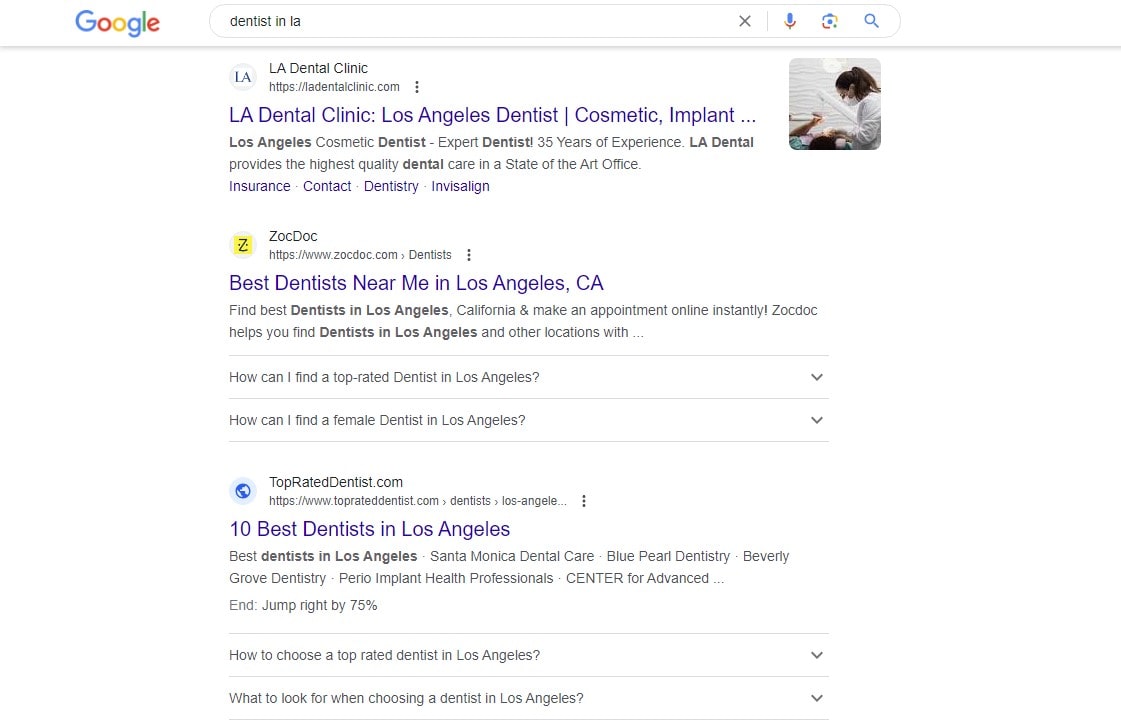The image displays a Google search results page with a clean, all-white background. At the top left corner, the iconic Google logo is presented in its standard multicolored lettering. Below the logo is a blank search bar where the query "dentist in LA" is typed. To the right of the search bar, there is an 'X' button designed to clear the search query, followed by three additional icons: a microphone for voice search, a checkerboard-like square, and a magnifying glass symbolizing the search function. A light gray line spans horizontally beneath this section, demarcating the search results.

The search results are shown underneath this gray divider, featuring three different dental clinic listings. Each result starts with a small circular icon or logo on the left side, followed by the name of the clinic or website highlighted in purple. Below the name, the web address is displayed in black text, along with a brief description.

The first result is for "LA Dental Clinic," with the title "Los Angeles Cosmetic Implant." Adjacent to this listing on the right is a square image depicting a woman in a white coat with her hair tied in a ponytail, seemingly engaged in a dental procedure.

The second result appears to be for "ZocDoc," identifiable by the name displayed prominently.

The third result mentions a site for top-rated dentists, focusing on dental services in an advertorial format.